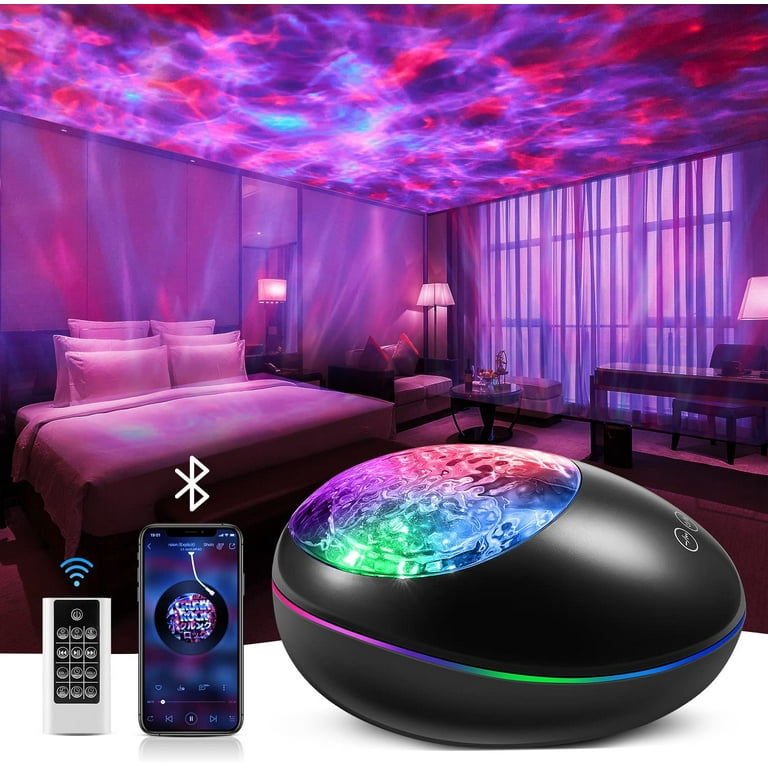This image is an advertisement for an innovative ambient lighting device designed to transform an entire room into a vibrant, multi-colored environment. The focal point is a large, sleek, egg-shaped device equipped with a translucent insert, which emits an array of programmable colors. This device can project these colors onto the walls, ceiling, and floor, creating a mesmerizing atmosphere. In the lower-left corner of the image, a remote control is displayed, illustrating one method of controlling the device. Additionally, the image highlights a complementary smartphone application that allows for seamless customization of lighting effects. Users can easily select their desired colors, adjust light patterns, and control the intensity—offering endless possibilities to personalize and enhance any space with dynamic lighting.